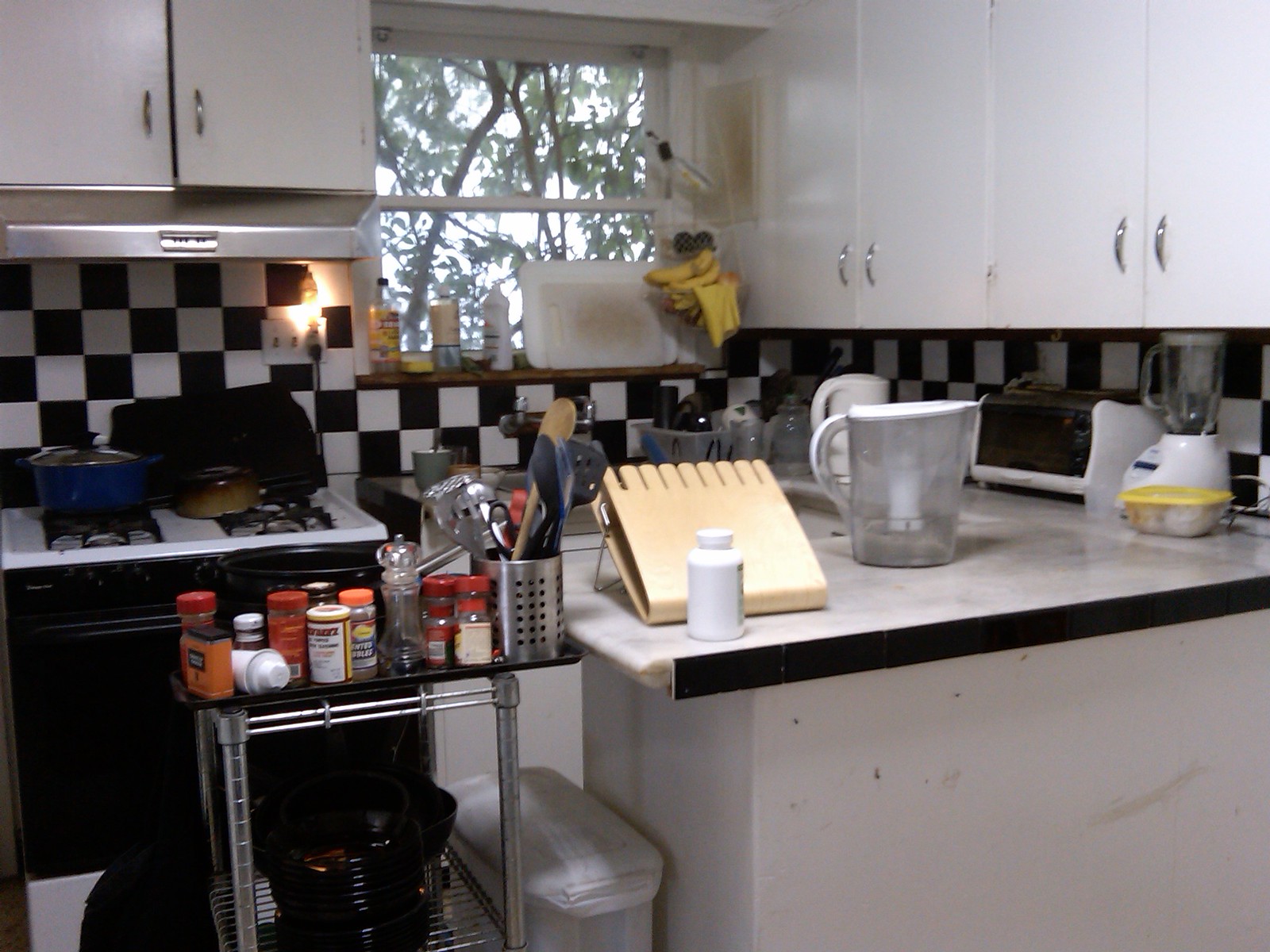A cozy home kitchen is depicted in this image. Dominating the background from the top left are two adjacent cabinets, beneath which hangs a sleek, chrome or stainless steel vent hood. Below the vent hood is a contrasted gas stove featuring a white top and bottom drawer, with the central oven section in black. The wall behind the stove displays a classic black and white checkered tile backsplash, extending around a corner to another wall on the right.

To the right side of the stove, a white countertop and a sink with shiny chrome fixtures are visible. Above the sink, a window filled with everyday kitchen items, including dish soap, cutting boards, and a hanging basket with bananas, adds a touch of homeliness. 

Further to the right, white cabinets are noticeable, and the countertop below them reveals a white or light gray marble pattern. Below this countertop appears to be a white base. 

In the left forefront of the image, a stainless steel rack or cart with a black top stands, laden with an assortment of spices, utensils, and a pot. Below the cart are several bowls stored neatly. A white trash can is situated between the counter and this cart, completing the scene.